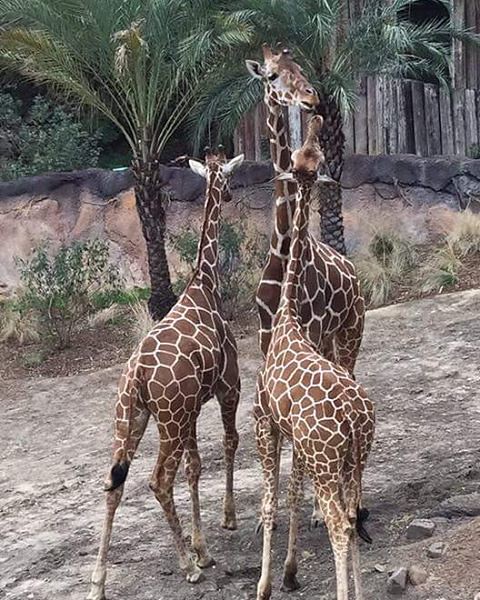In a naturalistic enclosure with a rugged, rocky surface, three giraffes stand grouped together. The setting features a sturdy stone wall interspersed with rustic wooden slabs forming a rustic fence, behind which additional bushy vegetation and palm trees, with scaly trunks and lush green fronds, reach upwards. The tallest giraffe, an adult, faces the camera while looking slightly to the right. In front of the adult, two smaller, juvenile giraffes stand with their backs partially turned to the camera, as though engaging with each other or being fed by the adult. The giraffes sport classic patterned coats of tan patches bordered by white, and the enclosure, complete with sparse, dry, and green shrubbery, contributes to a naturalistic, outdoor scenery.